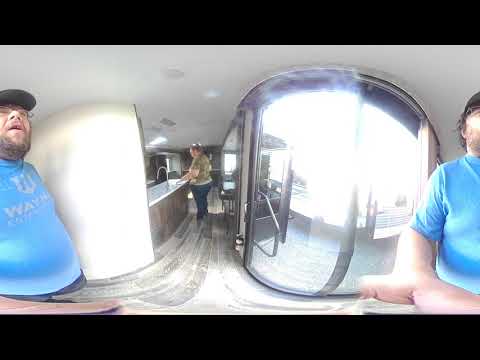This horizontally aligned, rectangular image features a thick black border at the top and bottom with a slightly blurry quality. It appears to have been taken indoors, potentially within a home. The image, exhibiting a 360-degree effect, might seem fragmented, but the left and right sides form a continuous panorama.

The scene is framed by a white or light gray ceiling, with a prominent, large curved or concave window centrally to the right, hinting at an outdoor view obstructed by the indoor focus. Behind the window, railings are faintly visible. A noticeable man appears twice, embodying the 360-degree effect. On the right side, we see part of his body in a blue t-shirt, with his ball cap-clad head turned upwards. On the left side, more details reveal his bearded face, rimmed glasses, and blue shirt with white print, notably the word "Wayne."

In the middle ground stands a woman dressed in jeans and a short-sleeved camo shirt, engaged with a large sink island featuring a curved faucet. She is washing something, looking downward. Additional details include a sliding glass door and some light fixtures, adding depth to the indoor setting embellished with a palette of off-whites, light blue, and tan hues. The overall ambiance suggests a casual, everyday moment captured in a slightly disorienting, panoramic format.